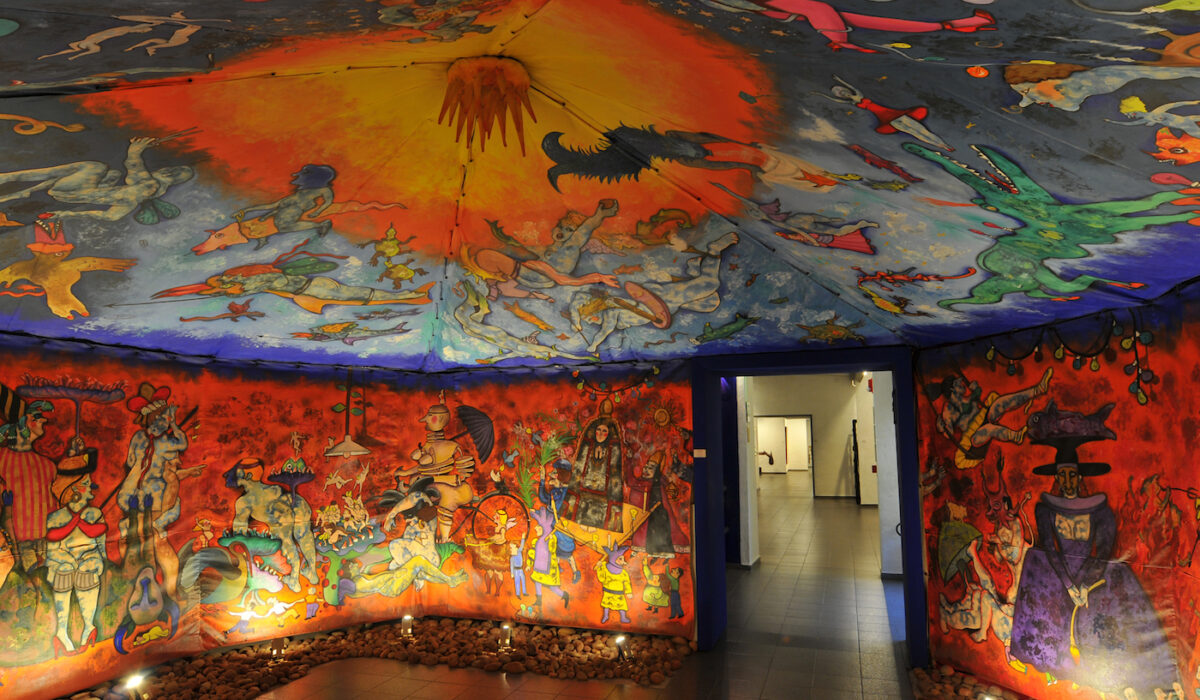The image depicts an elaborately painted oval room with a dome-like ceiling, adorned with a myriad of bizarre and intricate murals. The primary background color within the room is a vivid red, providing a canvas for various primitive and oriental-style caricatures. Among the notable figures, there is a woman in a long robe, a stylized person riding a bike with an umbrella, and several characters who seem to be clapping or involved in other strange actions. One particularly odd figure appears to be leaning over with something emerging from their rear end. 

On the right side, a witch-like figure with a broad black hat, clad in a purple gown and holding a golden rope, stands out. Above her, there is a green creature with its mouth open. The ceiling features an array of fantastical creatures, seemingly floating as if in water, with one that resembles a person riding an elephant or an alligator. The center of the ceiling is dominated by a striking yellow splotch, possibly representing the sun, with what looks like dripping fire emanating from it. Between the walls and ceiling, a purple lining divides the two areas.

The flooring is a brown stone, and there are rugs positioned in front of the murals, with lights illuminating the walls. In the bottom right corner of the image, an open doorway leads to a regular hallway with white, unadorned walls, suggesting that the setting might be an art gallery or an installation within a more conventional building. The room is brightly lit with ample natural light, enhancing the clarity and vividness of the surreal, cartoon-like imagery that covers nearly every surface.